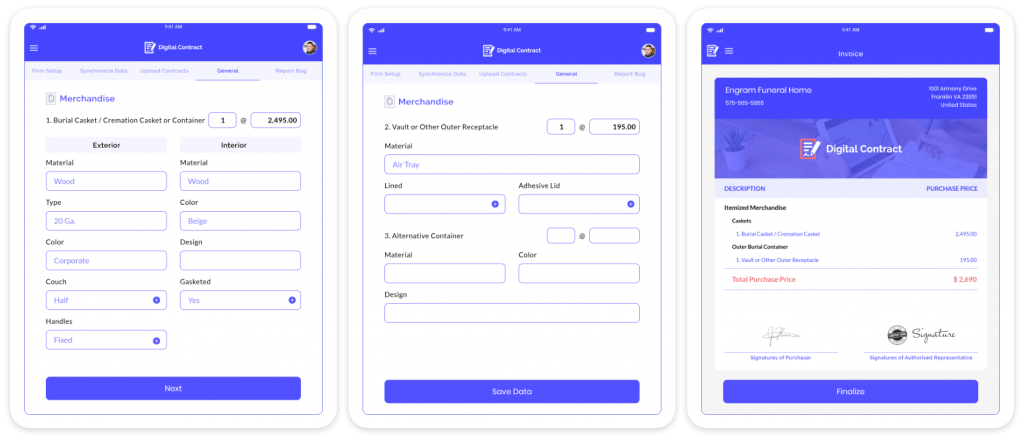This screenshot features a triptych of panels from an app, illustrating a detailed progression through various customization options for funeral merchandise. The first panel is under the 'General' tab, specifically labeled 'Merchandise.' Listed items include a burial casket and a cremation casket or container, each priced at $2,495. Users are able to personalize both the exterior and interior of the caskets. For the exterior, available options include the material (currently set to wood), type (20GA), and color (corporate color), with additional settings for the style of the couch (half) and fixed handles. The interior customization options allow for selecting materials (also wood), the color (beige), and include a setting for gasketed options (selected as 'yes') while the design field remains blank.

In the second panel, the focus shifts to the 'Vault and Other Outer Receptacle' section, where an item is selected at $195 with the material chosen as 'air tray.'

The third panel consolidates the total cost of the selected items from the previous panels, providing a comprehensive view of the final expenditures.